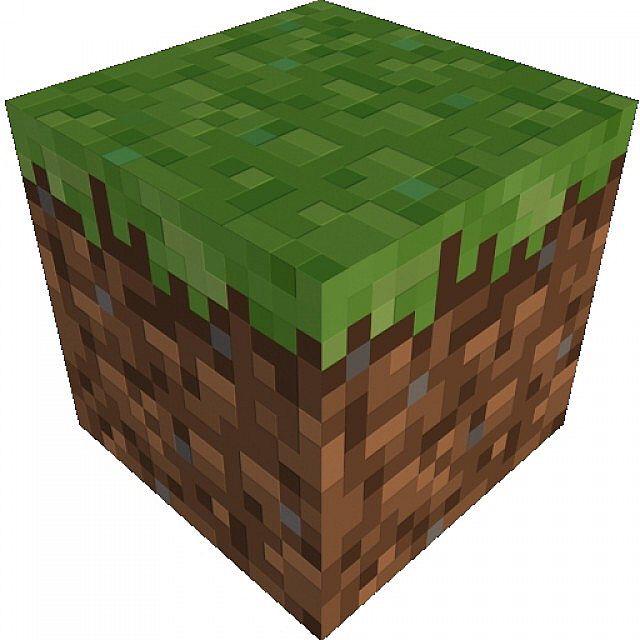The image features a three-dimensional Minecraft dirt block, characterized by its familiar pixelated texture. The lower portion of the cube, comprising approximately 80% of the block, mimics the appearance of soil with a detailed mix of light brown, dark brown, and medium brown pixels, interspersed with occasional bluish-gray dots. The upper portion, making up about a fifth to a quarter of the block, showcases a grassy layer rendered in various shades of green—light, medium, and dark—that spills slightly over the edges onto the brown soil beneath. The intricate pixel arrangement mimics the design's iconic look, making it instantly recognizable as a block from the Minecraft game. The perspective shows the corner of the block, enhancing its three-dimensional, computer-generated appearance.